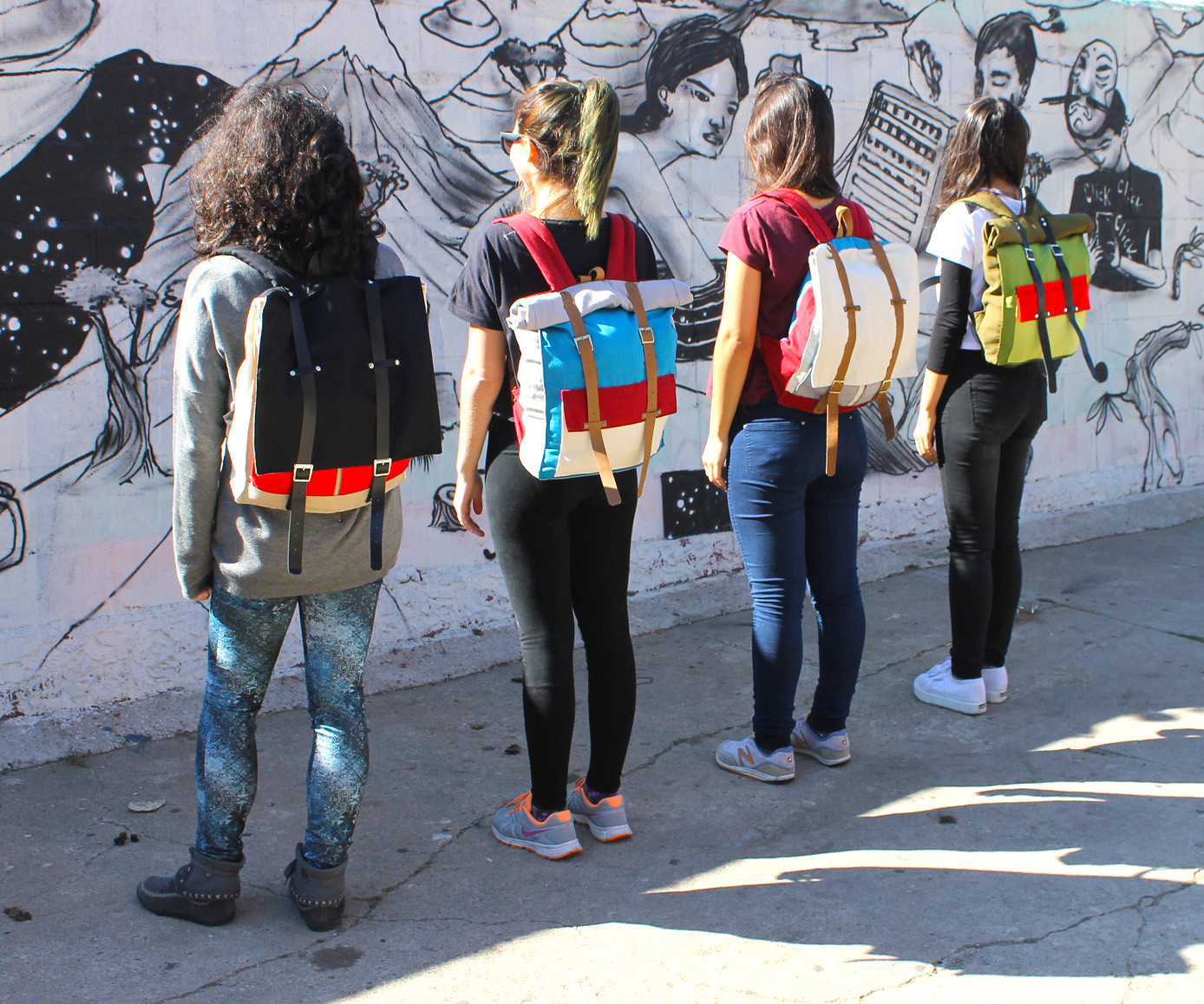This is an outdoor color photograph taken on a sunny day, depicting four high school-age girls standing in front of a wall adorned with an intricate black and white mural. The mural features a variety of detailed elements, including a night sky with stars, trees, mountains, and several faces and masks—one of which resembles a man with a mustache, reminiscent of a Salvador Dali mask. A notable section includes a woman and a couple of children.

The girls are arranged from left to right, their backs predominantly facing the camera, with slight three-quarter views. They are dressed casually in garments typical of school attire—jeans or leggings, sneakers, hoodies, and sweatshirts. Each girl is carrying a distinct, colorful backpack, possibly from the brand Quattro Paxi, featuring various fastenings and designs. The girl on the far left has dark curly hair, the next has blonde hair tied in a ponytail, followed by a girl with short brown hair, and lastly, one with darker brown hair.

They stand on a surface of broken macadam, casting shadows to the right due to the sunshine, observing the mural with intent. The setting suggests they might be part of a school group or tour, engrossed in the street art's captivating details.